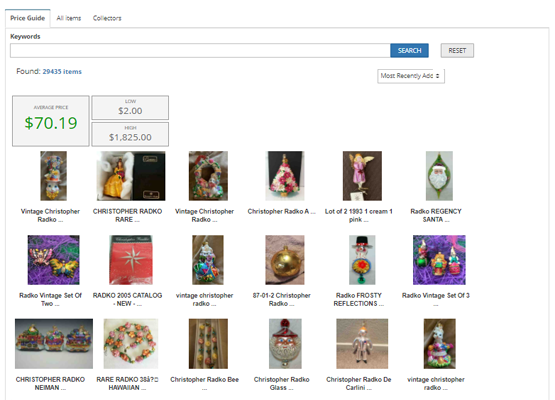This image depicts a webpage dedicated to a price guide, specifically for collectible items. The active tab is labeled "Price Guide," with additional tabs titled "All Items" and "Collect Tours" available for navigation. Directly beneath these tabs, there is a search box designed for keyword input, accompanied by a "Search" button to the right, and a "Reset" button further to the right.

The page indicates that there are a total of 29,435 items found. Below this information, there is a section labeled "Most Recently Added." On the left side of this section, there is a box displaying a price of $70.19, with two smaller boxes underneath it showing a price range: "Low $2" and "High $1,825."

Further down, the webpage showcases 18 images laid out in a grid format, each pertaining to various Christopher Radco collectibles. The detailed descriptions for each item from top to bottom, left to right are as follows:

1. Vintage Christopher Radco
2. Christopher Radco Rare
3. Vintage Christopher Radco
4. Christopher Radco A
5. Lot of two (1993): One Cream, One Pink
6. Radco Regency Santa
7. Radco Vintage Set of Two
8. Radco 2005 Catalog New
9. Vintage Christopher Radco
10. 87-01-2 Christopher Radco
11. Radco Frosty Reflections
12. Radco Vintage Set of Three
13. Christopher Radco Newman Rare
14. Radco 324 Hawaiian
15. Christopher Radco B
16. Christopher Radco Radio Glass
17. Christopher Radco De Carlini
18. Vintage Christopher Radco

Each item appears to be distinct and collectible, characterized by relevant names and details conducive to a collector’s search for specific Christopher Radco pieces.